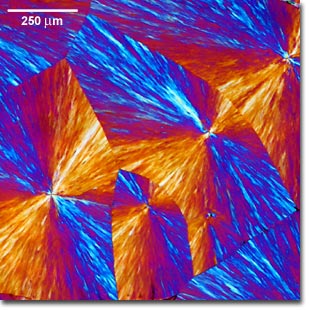This image features a vibrant piece of rendered artwork showcasing a dynamic interplay of electric blue, orange, and hints of white. The composition is marked by abstract arcs filled with sprays and streaks of these vivid colors, creating a fan-like, triangular geometry. Intricate details reveal light blue streaks within the blue sprays, and white streaks intertwining with the orange. In the top-left corner, a white bar line is present with the text "250UM" also in white. This computer-generated artwork gives a futuristic impression, with its kaleidoscopic patterns and square-shaped panels blending seamlessly to evoke a sense of scientific or cosmic exploration. The piece is detailed and complex, pairing geometrical precision with an organic flow, potentially symbolizing an advanced digital creation.